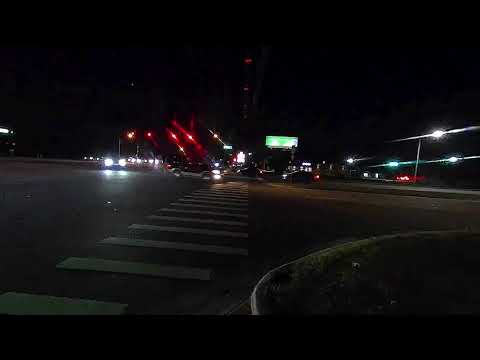This nighttime photograph captures a dimly lit city intersection, characterized by a broad crosswalk in the foreground that stretches across the street. On the left side of the crosswalk, a car is visible making a left turn, while additional vehicles, their headlights prominent, approach the intersection. To the right, there are more vehicles with their taillights glowing. The scene is framed by various lights and buildings, though the structures aren't notably tall. In the distance, directly ahead, a large building or tower rises against the pitch-black sky. Several red and white lights illuminate the area, and a conspicuous green road sign, potentially a navigation or billboard sign, can be observed in the center of the image. The overall mood is marked by the sparse illumination typical of an urban nightscape.